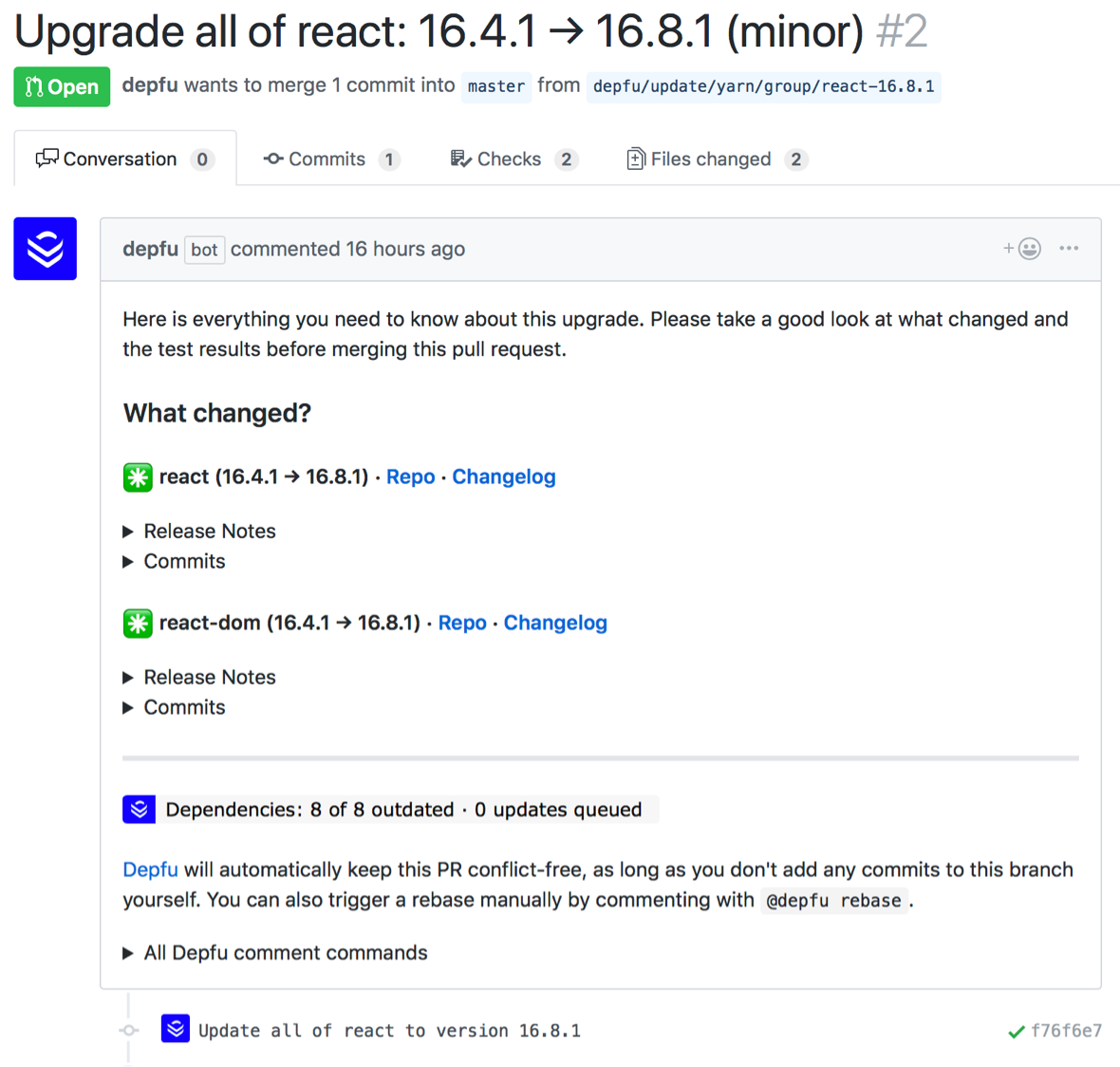A screenshot of a GitHub webpage showcases a pull request titled "Upgrade all of React from 16.4.1 to 16.8.1." The request has been initiated by the user Depafu, who seeks to merge one commit into the master branch. The page is predominantly white with minimal, colorful accents, typically associated with GitHub's interface.

A comment from Depafu Bot, made 16 hours ago, stands out, offering a detailed explanation of the upgrade process. The bot advises reviewers to examine the changes in the test results before proceeding with the merge, emphasizing the importance of ensuring stability and functionality. 

The page includes technical details commonly understood by programmers and engineers, such as sections labeled "Release Notes," "Commits," and information about dependencies, noting eight outdated dependencies with no updates currently queued. This specialized jargon can be intimidating to those not well-versed in computer science but is second nature to professionals in the field.